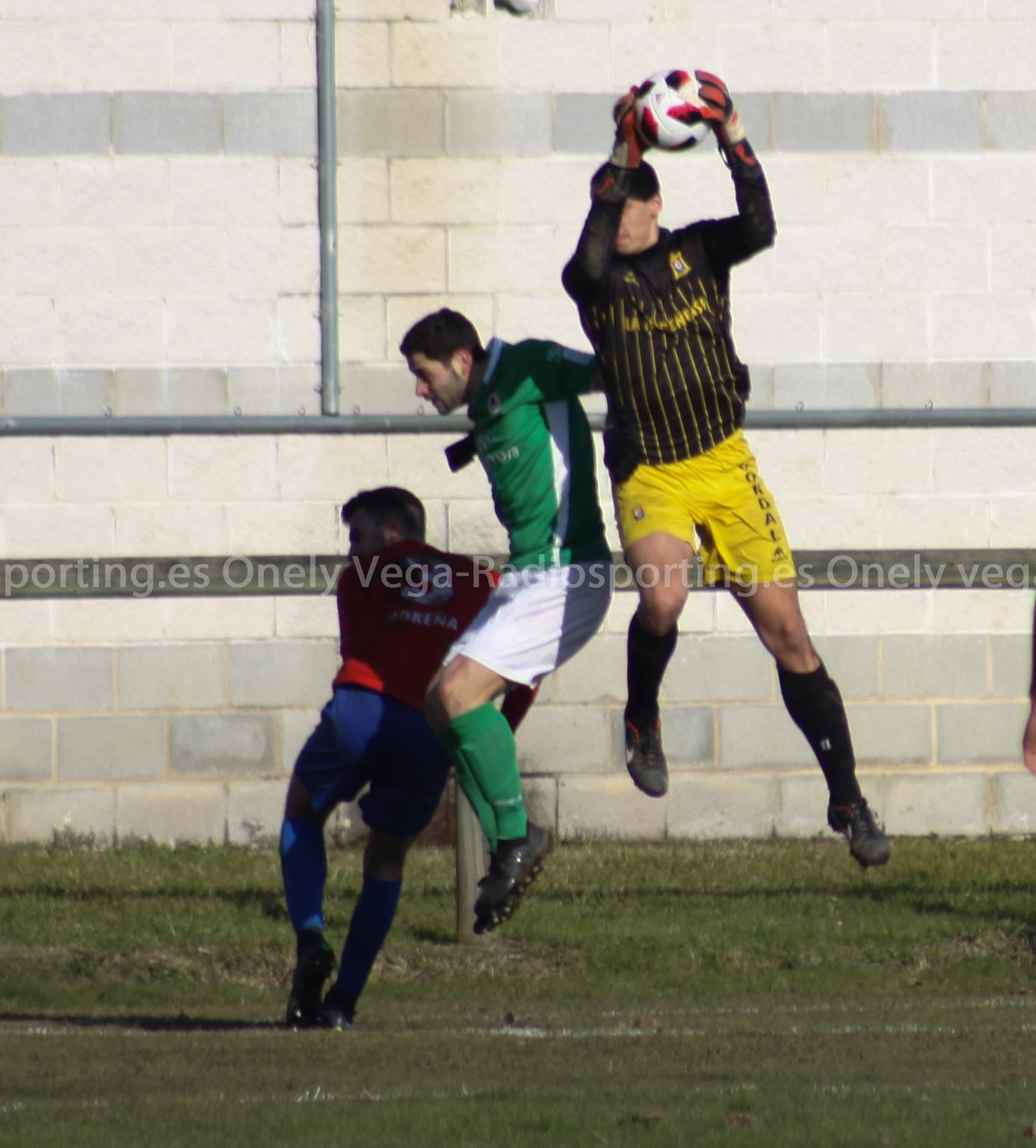The image is a rectangular, almost square outdoor photograph capturing a dynamic moment in the middle of a soccer game. Set against the backdrop of a white cinder block wall, the game is in full swing on a lush green grass field. Three players, each in distinct uniforms, dominate the scene. The central figure, clad in a black and yellow uniform with yellow shorts and black socks, is airborne, clutching the ball. To his immediate right, also mid-air but facing away, is a player in a white, green, and black uniform. On the ground, with his back to us, the third player wears a red and green outfit. Except for the players, the field is empty of other people. A horizontal banner across the image displays text that reads "Only Vega Radiosporting.es," repeated uniformly for advertisement.